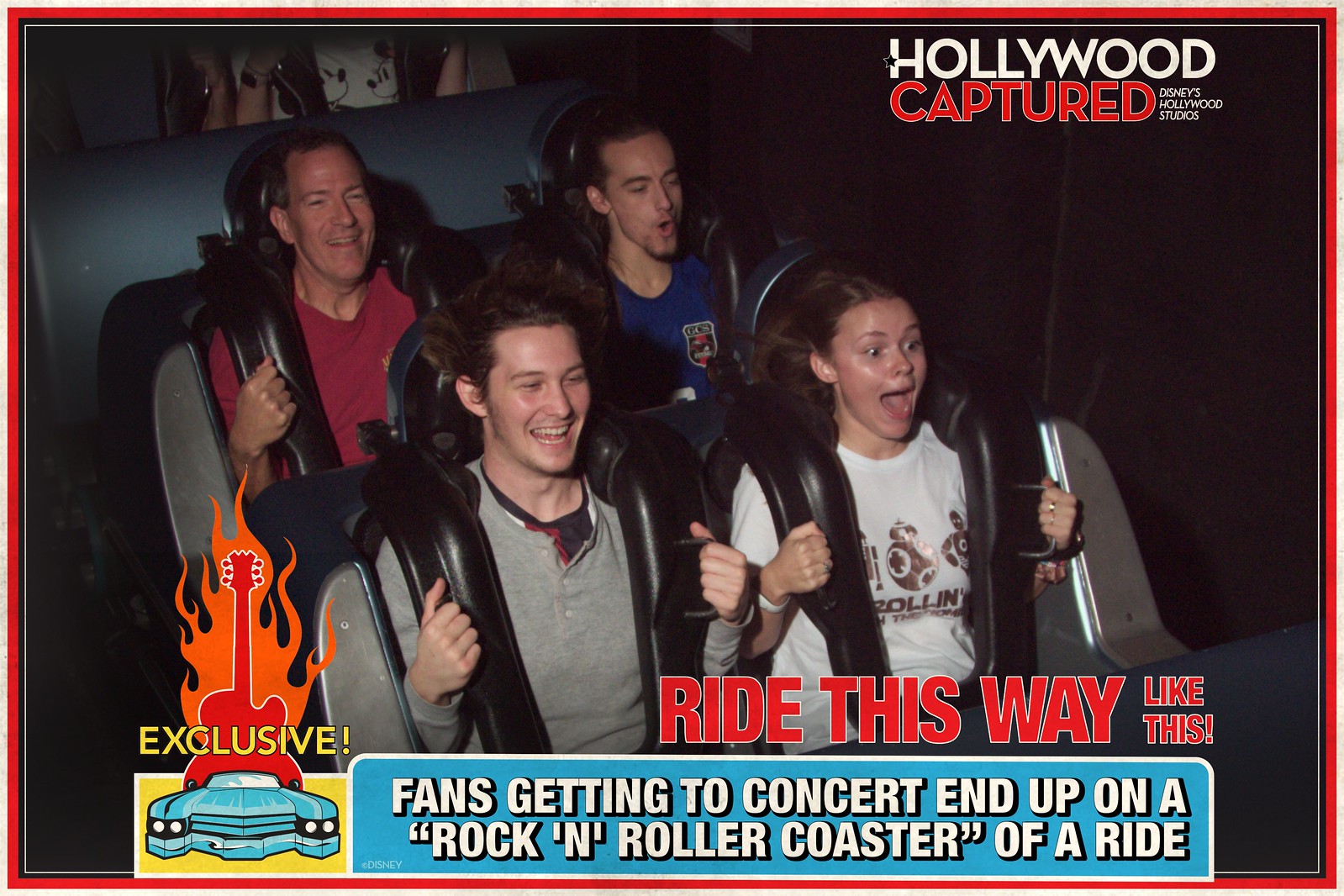Set against the dimly lit backdrop of Disney's Hollywood Studios, a vivid snapshot captures the thrilling moment on a Rock 'n' Roller Coaster. In the front row sits a young girl in a white shirt, her face a mask of exhilaration, tightly secured by a black shoulder harness. Beside her, a man in a gray long-sleeved shirt shares the same type of restraint, his expression a fusion of excitement and laughter. Behind him, a man in a red shirt mirrors his thrill, while another man in a blue shirt, seated behind the girl, completes the quartet. Above them, the words "Hollywood captured" stand out, with "Hollywood" in white and "captured" in red, amidst the dark atmosphere of the ride. A vibrant advertisement at the bottom features a blue car driving forward, a flaming red guitar, and the bold proclamation "Exclusive." Additional text within a blue box declares, "Fans getting to concert end up on a rock and roll rollercoaster of a ride," encouraging viewers to "ride this way!" This dynamic image encapsulates the intense joy and adventure synonymous with theme park thrills.